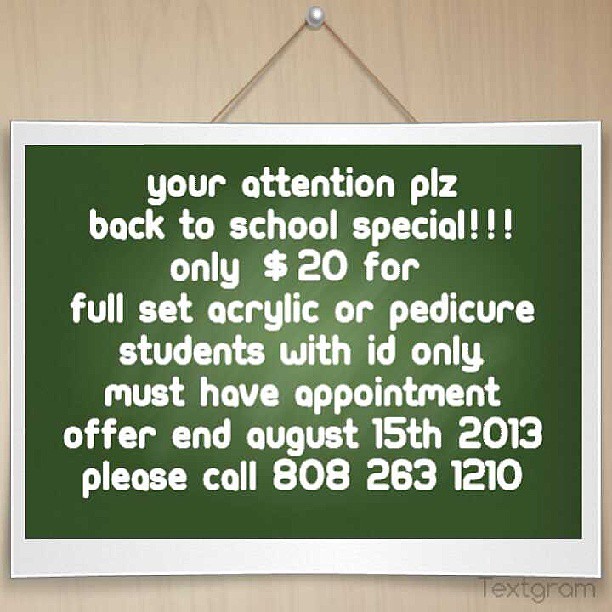The image depicts a promotional sign for a pedicure business, set against a light brown background that resembles a wall. A round white thumbtack secures a string in a triangular shape, suspending the sign. The sign itself features a green background surrounded by a white border. 

The text on the green background is in white and largely centered, using a consistent digital font, all in lowercase. The sign prominently reads, "your attention plz back to school special!!!", advertising a $20 offer for either a full set of acrylic nails or a pedicure, exclusively for students who present a valid ID. It specifies that appointments are necessary and notes that the offer ends on August 15, 2013. The sign provides a contact number for bookings: 808-263-1210. In the bottom right-hand corner of the image, the word "Tex-Gram" is subtly displayed in dark, lightweight font.